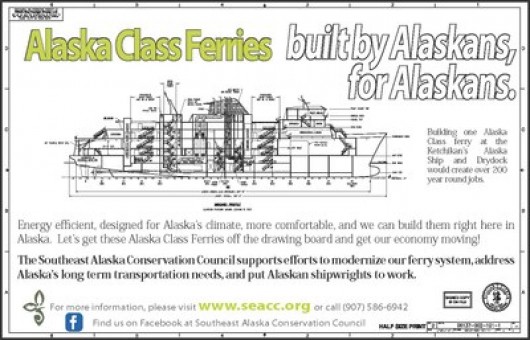The image features an advertisement for Alaska class ferries with a horse-lined rectangular frame and a black border. In the upper left, "Alaska Class Ferries" is written in a light or medium green color. To the right, a bold black-outlined white caption states, "Built by Alaskans for Alaskans." Below this, there is a black-and-white, somewhat blurry diagram of a ferry, with indistinguishable labels and numbers. Another caption explains that constructing an Alaska class ferry at Ketchikan's Alaska Ship and Dry Dock would create over 200 year-round jobs. Further down, text emphasizes the energy efficiency, comfort, and suitability of these ferries for Alaska's climate, urging to get them off the drawing board to boost the economy. At the bottom, bold black text notes that the Southeast Alaska Conservation Council supports modernizing the ferry system, addressing long-term transportation needs, and employing Alaskan shipwrights. For more information, visit www.scac.org or call 907-586-6942. Find the Southeast Alaska Conservation Council on Facebook.